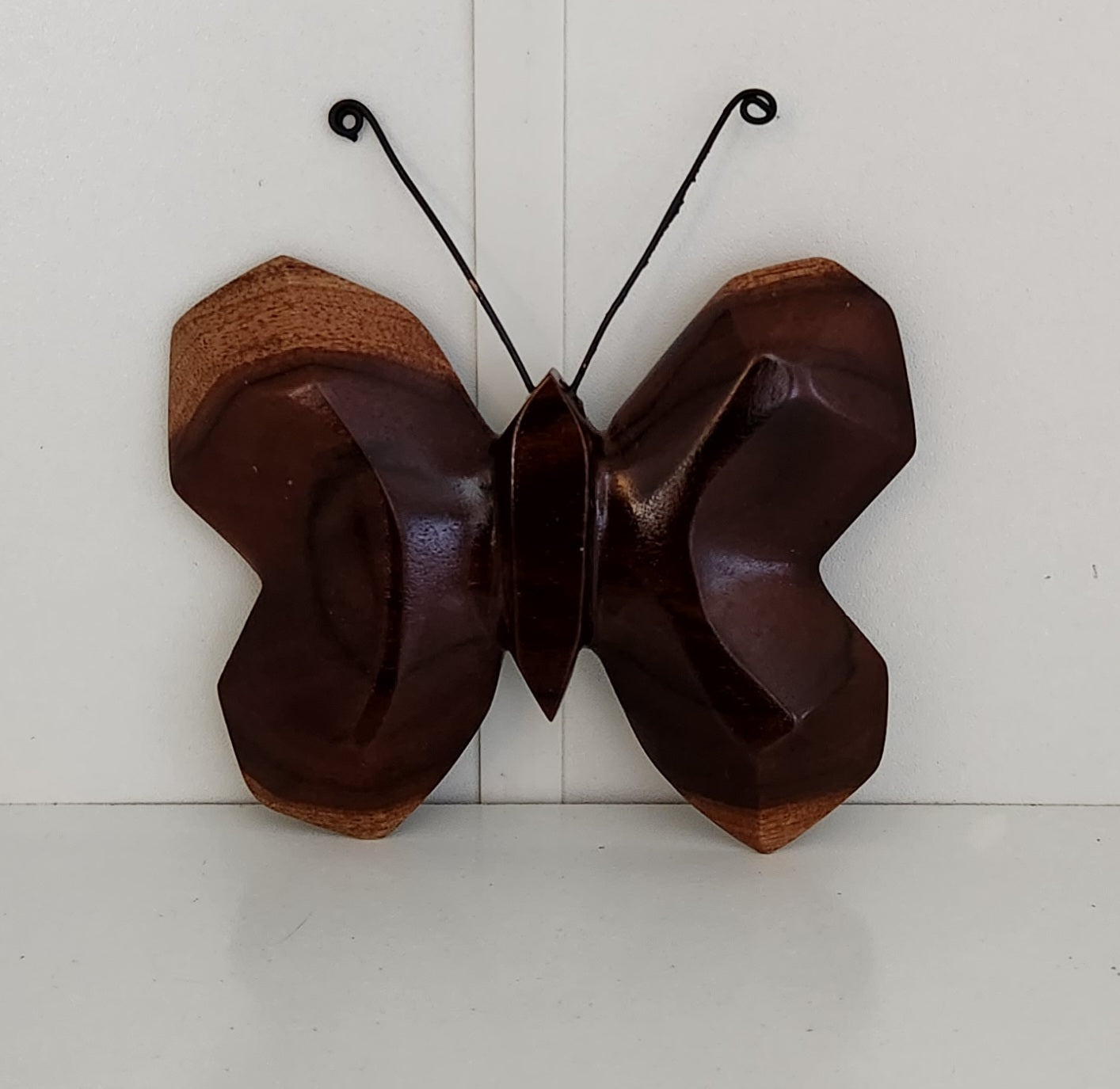This image portrays a detailed, color photograph of a large, sculpted butterfly art piece. The butterfly, expertly carved from dark brown wood with lighter, copper-hued accents, is mounted against a white wall. Its impressive wings, reminiscent of kidney beans and symmetrical in shape, display intricate craftsmanship with dark and lighter shades of brown, particularly notable at the tips. The central body is an elongated, tapered ellipse with a darker brown finish, adding to the lifelike aesthetics. Two metallic antennae, curled inward at the tips, project from its head, enhancing the sculpture's resemblance to a real butterfly. The piece rests on a white, shiny surface, reflecting some of the butterfly's features, adding depth to the artwork. The style is photographic realism, capturing the fine details and essence of the sculpture.